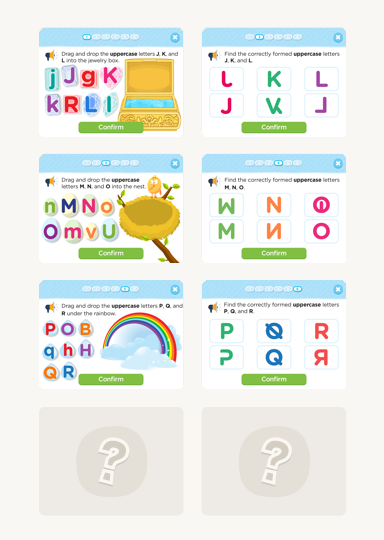This is a screenshot of a letter-based application interface. The main section features eight tiles, each displaying combinations of the letters "J," "K," "G," "R," and "L." These letters are arranged in various formats within rectangular boxes. The tiles are presented in different colors and layouts, creating a diverse visual display. The bottom row of tiles contains gray question marks, indicating incomplete or hidden elements. The background of the interface is white, and a distinctive blue bar runs across the top of the screen. Overall, the purpose and functionality of the application remain unclear from this image.